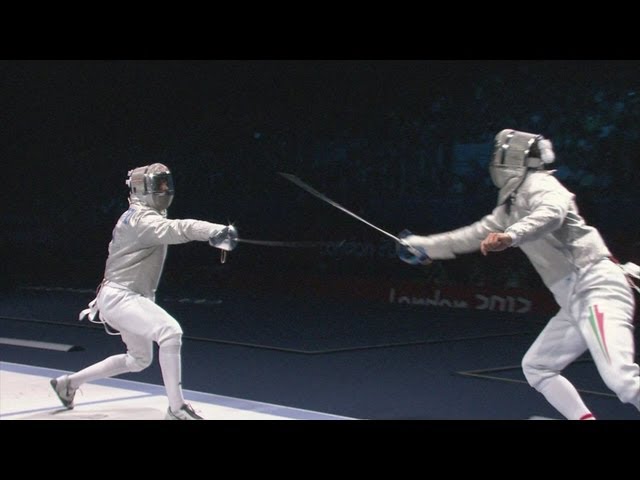This captivating black and white photograph captures a dramatic moment from the London 2012 Olympics fencing event. Two fencers in motion are locked in intense combat on the fencing piste. The fencer on the left, in a semi-crouched defensive stance with his right arm and fencing foil fully extended, appears to be bracing for an attack. The fencer on the right, almost airborne, lunges forward aggressively, aiming his foil at his opponent. Both athletes are clad in traditional white fencing outfits, complete with protective helmets featuring metal mesh visors, and are wearing tennis shoes. The backdrop is largely dark, shrouding the audience in obscurity, but a partially visible red banner with the text "London 2012" identifies the prestigious setting of this exhilarating face-off.